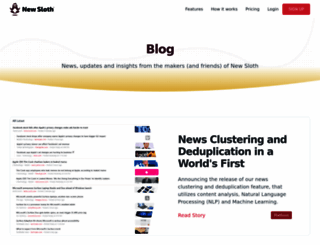An image is displayed with a predominantly white background and black text. At the top left corner, the text reads "New Sloth" which could indicate a new update or feature. The main image showcases an animal that seems ambiguous; it could be misconstrued as either a sloth, which is referenced, or a penguin based on its unclear appearance. Across the top menu, there are several navigation links including "Pricing" and "Login," followed by the label "Blog."

On both the left and right sides of the image, there are additional links. To the right, there is a notable heading: "News Clustering and Deduplication in a World's First," accompanied by some explanatory text, though its details are not fully visible. There is a red button located at the bottom right corner of the image whose text remains unreadable.

This image appears to be promoting a platform, potentially a blogging or news aggregation service that specializes in organizing and removing duplicate content, indicated by terms like "news clustering" and "deduplication." Overall, while the image layout is simple and primarily functional, the mixture of ambiguous imagery and scattered informative text gives it a somewhat cluttered appearance.